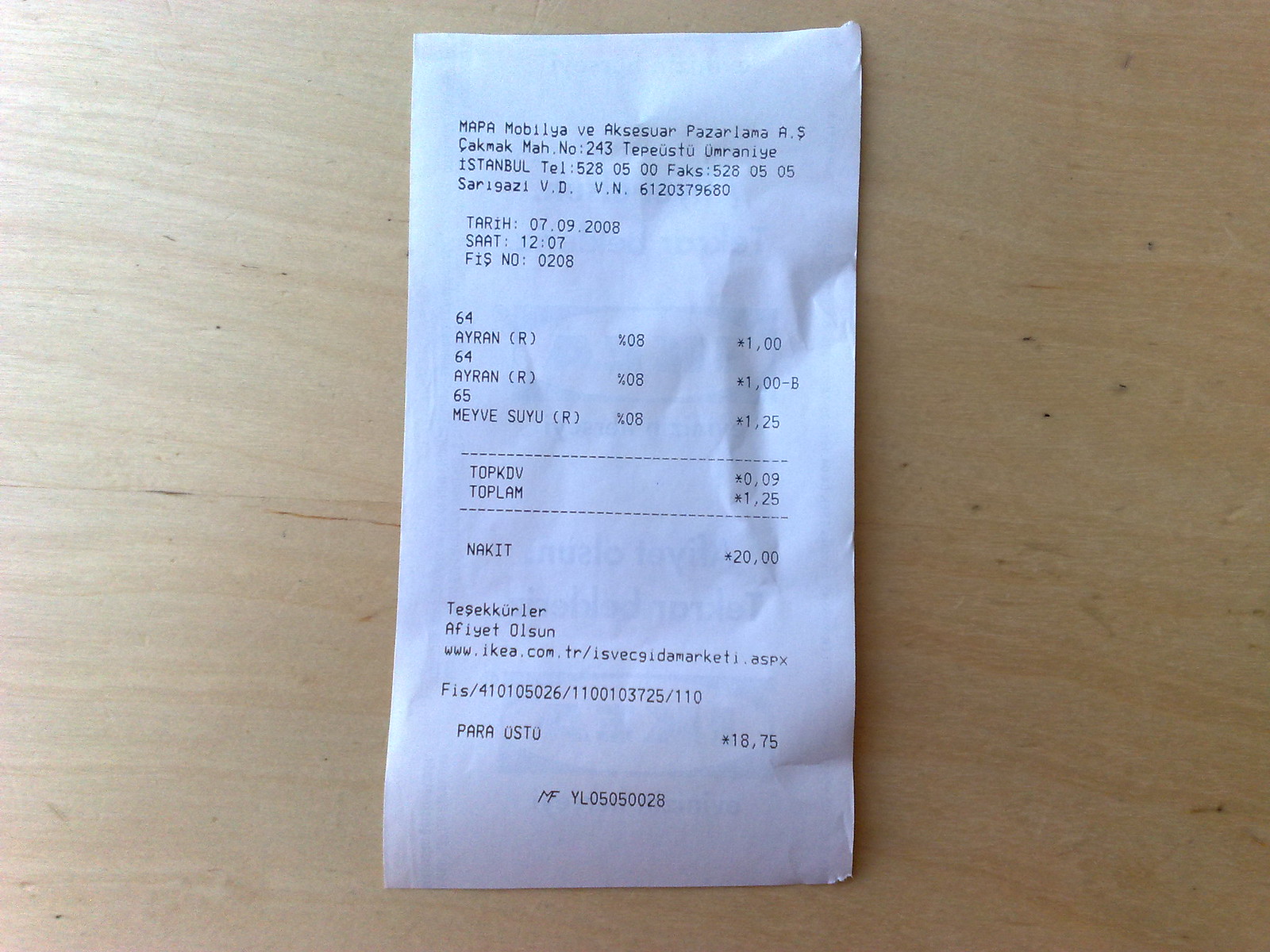The image displays a white paper receipt with black print generated by a computerized cash register. The receipt, written in what appears to be Spanish, includes detailed information about the purchased items and their respective prices. The listed items are:

1. **Ayran** (64 A-Y-R-A-N (R)) with a tax rate of 0.08%, priced at $1.00.
2. **Ayran** (repeat of the first item) with a similar pricing and tax rate indication: $1.00.
3. **Meyvesuyu** (65 M-E-Y-V-E-S-U-Y-U (R)), which also carries a tax rate of 8%, priced at $1.25.

In addition, the receipt shows:

- **TOP KDV**: indicating an additional taxation amount of $0.09.
- **TOP LAM**: summing up to a total of $1.05.
- **NAKIT**: with a cash payment amounting to $20.00.